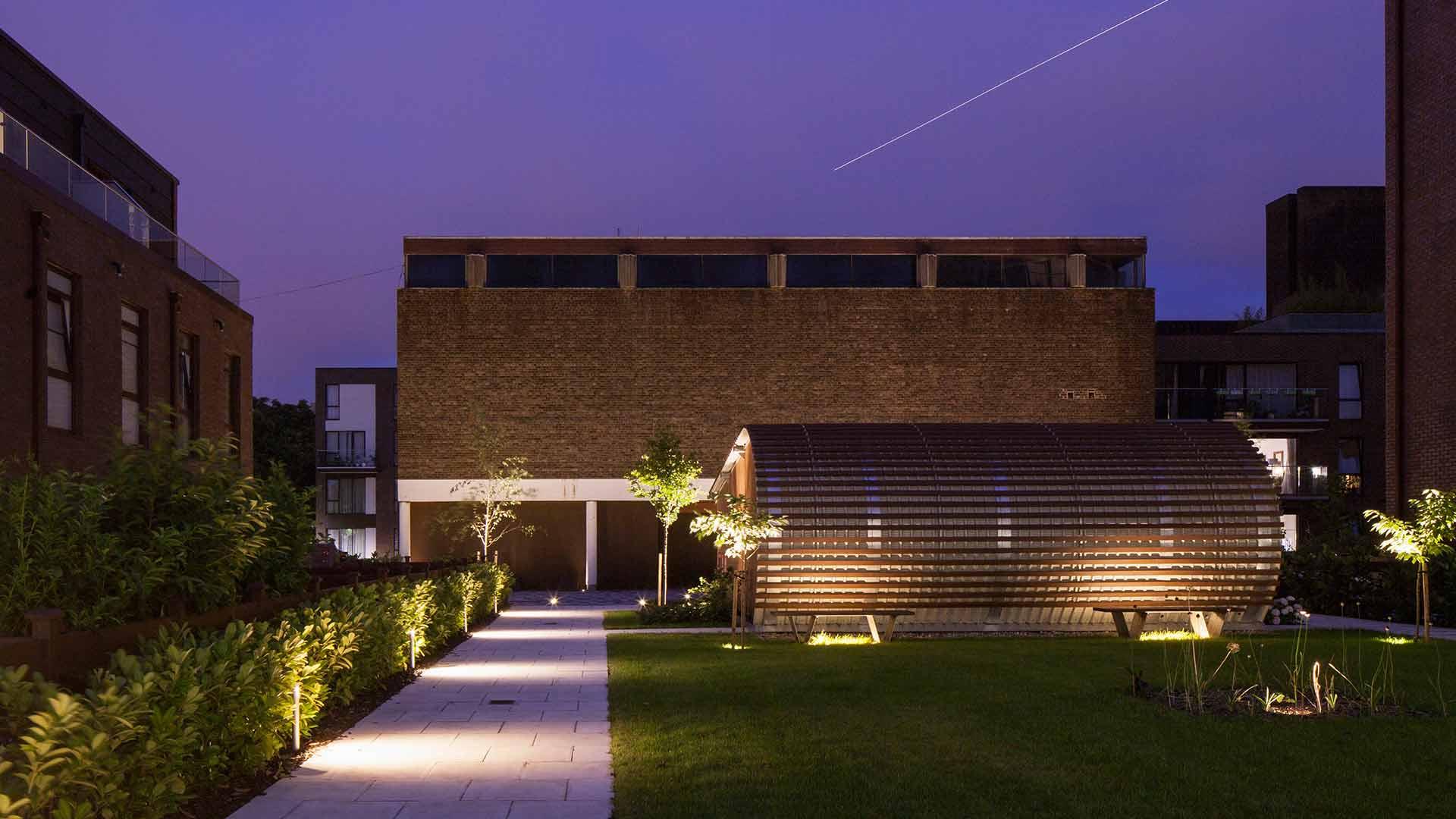This is an evening photo of an inside courtyard surrounded by brick buildings on three sides, with one in the foreground appearing modern despite its brick construction. The courtyard, illuminated subtly by post lights nestled within green bushes, features a stone pathway and a lawn area flanked by small trees and gardens. The buildings, which span two stories, have few windows, some of which are lit up, especially on the right-hand side. At the center of the courtyard, there's a cylindrical-shaped, arched structure, possibly a seating or covered area. Nearby, there are two benches and additional plant spaces with lights. The sky, transitioning from dusk to night, reveals a shooting star or the trail of an airplane, enhancing the serene and picturesque ambiance of what looks like a university campus.